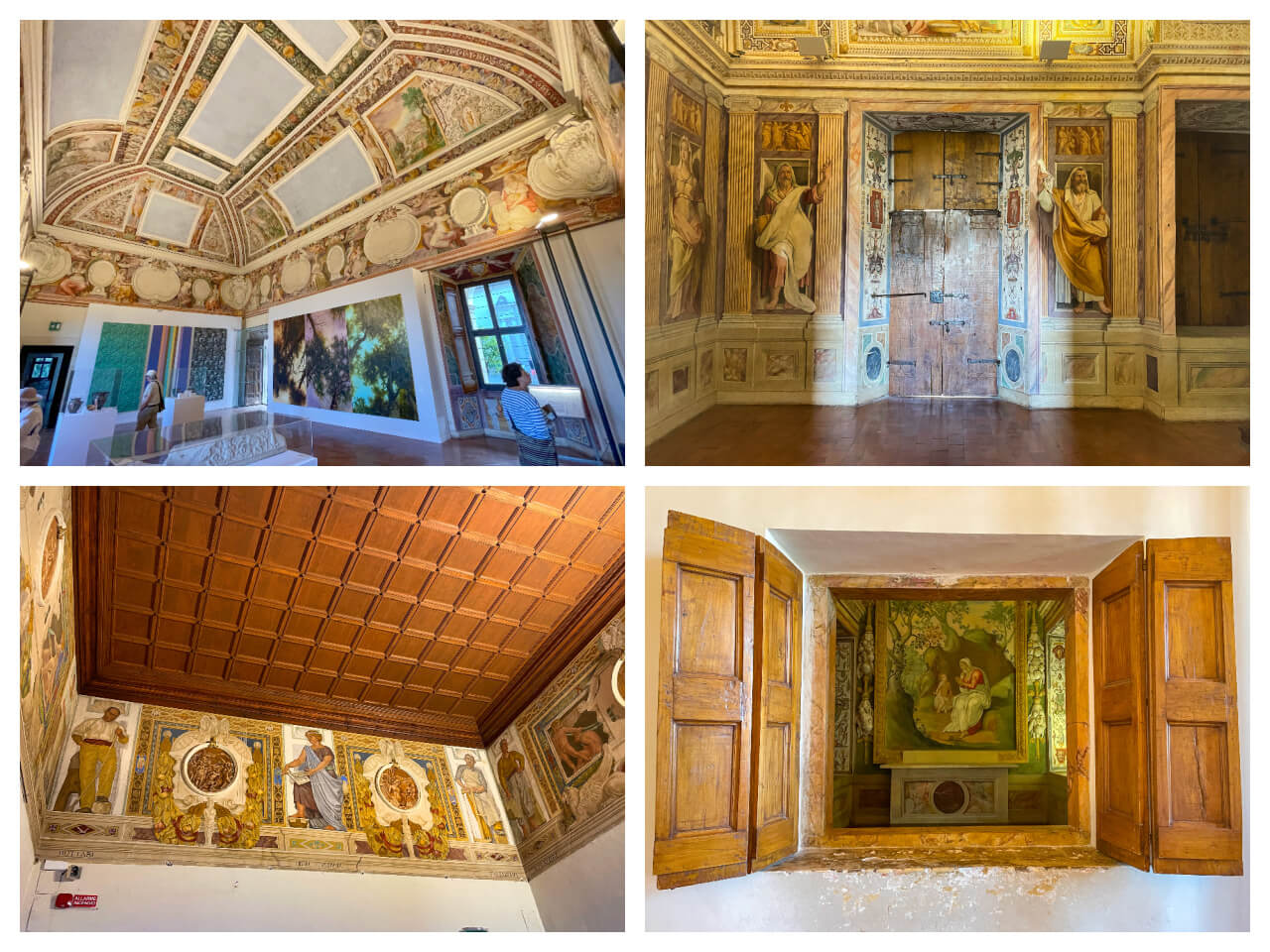This image is a composite of four equally-sized, landscape-oriented color photographs, arranged in a grid with white borders separating them horizontally and vertically. Each photo captures a different aspect of the same museum. 

The top left photograph offers an interior view of a grand room with an ornate domed ceiling and multiple oversized wall paintings. Scattered around the room are a few visitors admiring the surroundings. The top right image presents another section of the museum, focused on an entryway flanked by statues and vivid murals depicting standing figures. 

The bottom left photograph emphasizes intricate medieval and Greek mythological designs painted around a dark wooden ceiling with cross panels and raised wood details. Art paintings adorn the side walls, contributing to the rich aesthetic. The bottom right image showcases an exterior wall with open wood shutters revealing more artistic displays inside, alongside what appears to be wood shavings on the ground, suggesting recent carving work. Together, these images provide a detailed and immersive look into the museum's elaborate interior and exterior artistic elements.